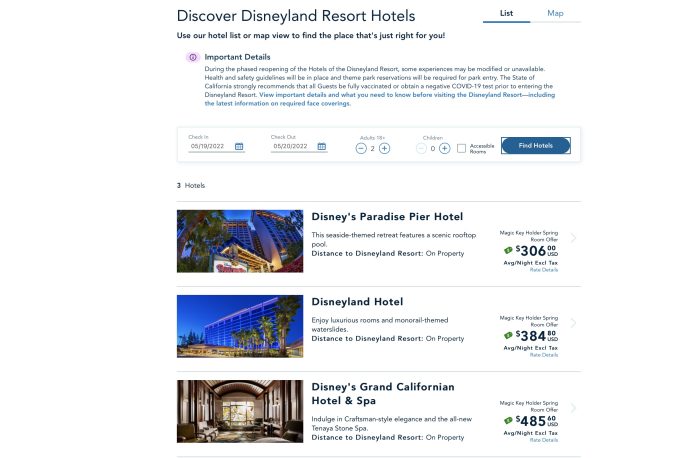The screenshot features a booking interface for Disneyland Resort Hotels set against a white background. Dominating the top of the screen in large black letters is the heading "Discover Disneyland Resort Hotels." To the right of this heading are two clickable headings: "List," which is in black and underlined in blue, and "Map," which is in blue.

Two lines below the main heading, in small black print, is the guidance text: "Use our hotel list or map view to find the place that's just right for you!" Beneath this line, there is a red icon followed by the bolded text "Important Details," under which are about five lines of smaller black text, with the last line highlighted in blue.

Further down, there's a horizontally elongated white rectangle outlined with a light blue line. This section allows users to input their dates of check-in and check-out, the number of adults, and other relevant details. To the right of this input section is a blue "Find Hotels" button.

Below this section, to the left, it states "3 Hotels" followed by a light gray line. Then there are three hotel listings, each consisting of a picture on the left, the hotel's name in the center, and the price along with additional details on the right. 

The first listing is "Disney's Paradise Pier Hotel," priced at $306. The second hotel is "Disneyland Hotel," priced at $384. The final listing is "Disney's Grand Californian Hotel & Spa," which is priced at $485.